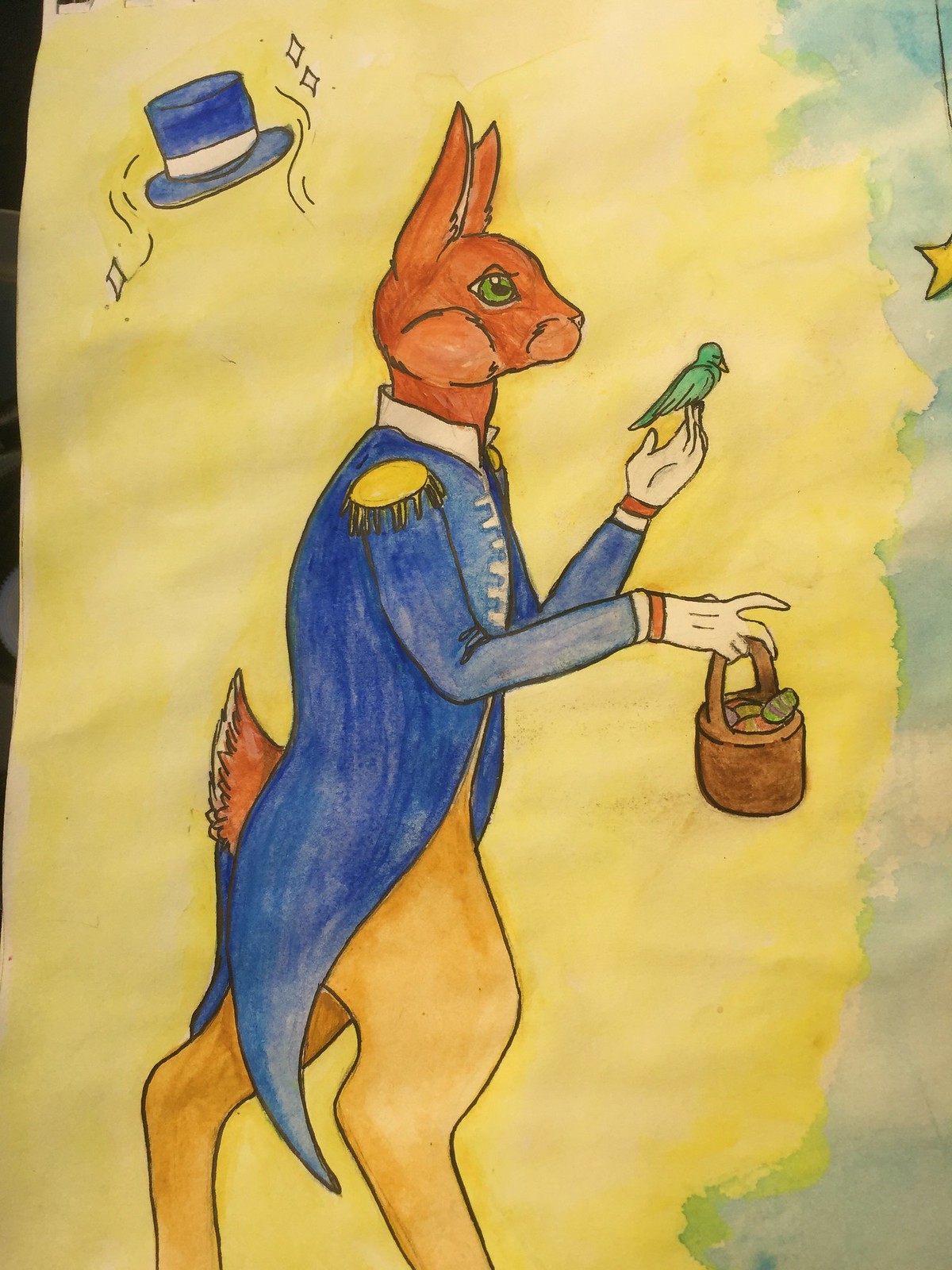In the center of the image is a detailed painting of a light brown rabbit standing upright on its hind legs, dressed in a blue military-style jacket adorned with yellow shoulder pads. The rabbit has striking green eyes and white gloves on its paws. It carries a small brown basket filled with Easter eggs in its right hand, while a small green bird perches delicately on the fingers of its outstretched left hand. The rabbit's blue top hat, decorated with white diamonds, floats just above and slightly behind its head. The background transitions from a yellow hue on the left, containing a small yellow star, to a gray shade on the right. The rabbit appears to be walking towards the left, looking ahead with a poised expression.